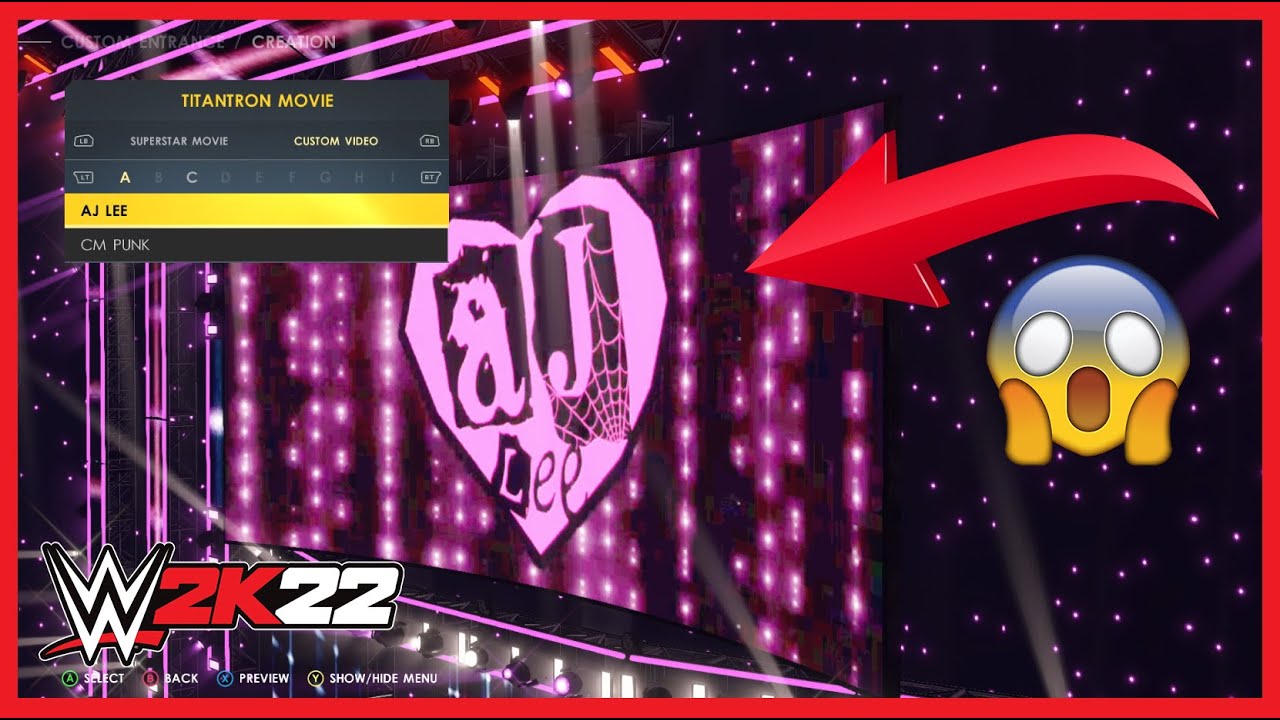This image is a detailed screenshot from what appears to be a WWE video game, specifically the WWE 2K22 series. The frame is bordered by a thin red line. In the upper left corner, text reads "Custom Entrance Creation" and below it, "Titantron Movie" is highlighted in yellow. The background of the interface is gray, featuring a large red arrow pointing towards the center where a rectangular screen displays the name "AJ Lee" in pink letters with a pink heart underneath it, emitting dramatic stage lighting effects. Below "AJ Lee," the name "CM Punk" is listed. To the right side, there's an emoji with its mouth open, eyes wide in white, and hands on its cheeks, illustrated with a yellow face and blue forehead, depicting a shocked expression. The bottom section of the image includes controls: the "WWE 2K22" logo in the bottom left, accompanied by buttons labeled "Select," "Back," "Preview," and "Show/Hide Menu."